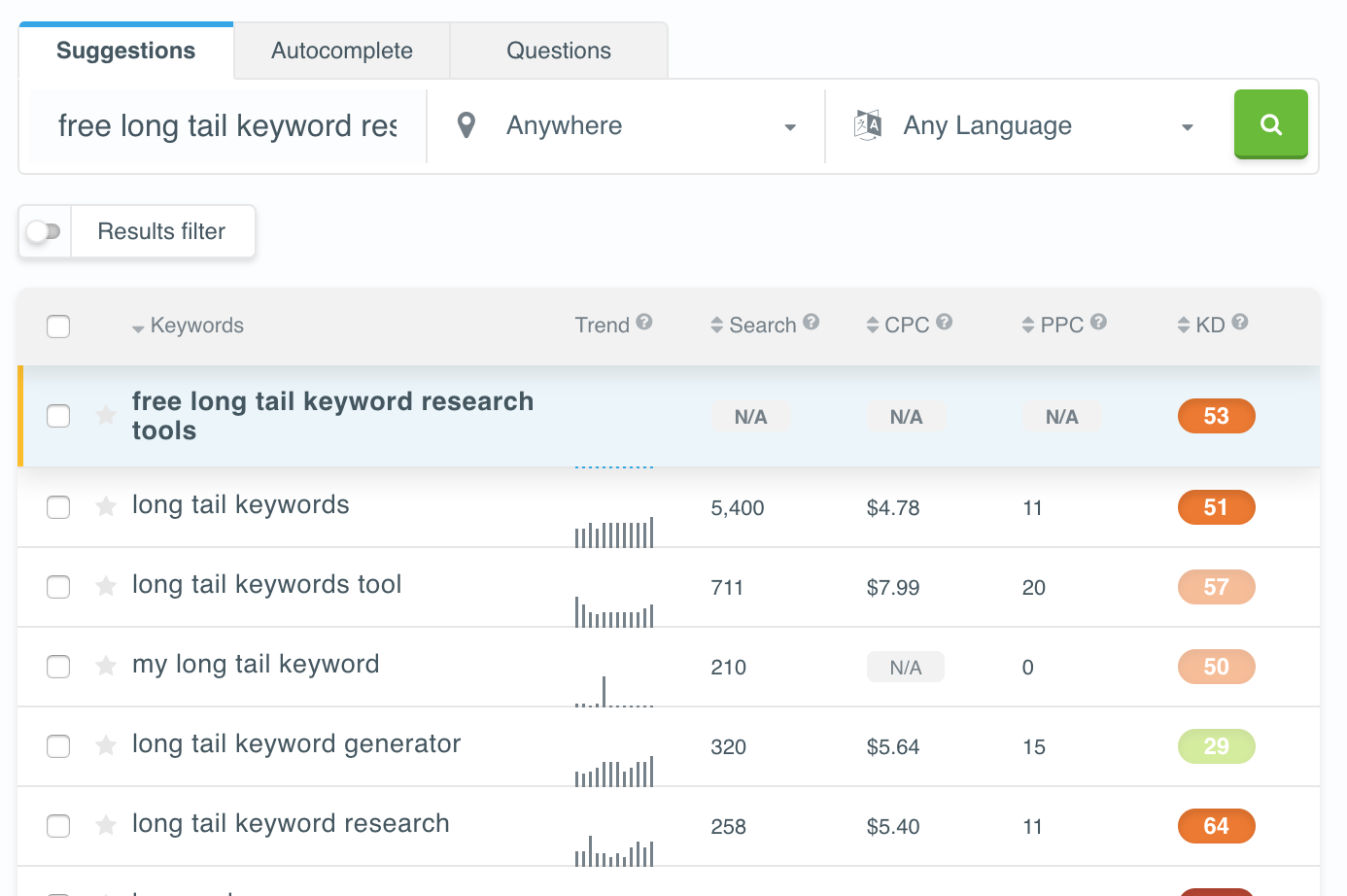This is a screenshot capturing a detailed view of an advertising metrics page related to keyword analysis. The interface displays three main tabs at the top, labeled "Suggestions," "Autocomplete," and "Questions," with "Suggestions" being actively selected, indicated by a white background and a blue underline, while the other two tabs are in gray.

The page’s background is white, maintaining a clean and minimalist design. Beneath the tabs, there's a search bar where the user appears to have partially typed "free long tail keyword," with the rest of the text truncated. Adjacent to the search bar, there are filter options displayed as drop-down menus labeled "Anywhere" and "Any Language," along with a conspicuous green search icon.

Directly below this search and filter area, a section to display results is evident, set up in a manner resembling a database table with multiple columns: "Keywords," "Trend," "Search," "CPC," "PPC," and "KD." The first result listed under the "Keywords" column is "free long tail keyword research tools," highlighted in blue. However, the associated columns for "Search," "CPC," "PPC," and "Trend" display as "N/A."

The page showcases six to seven keyword entries generated from the user’s search query, emphasizing the tool's role in providing keyword suggestions and associated metrics for advertising purposes.